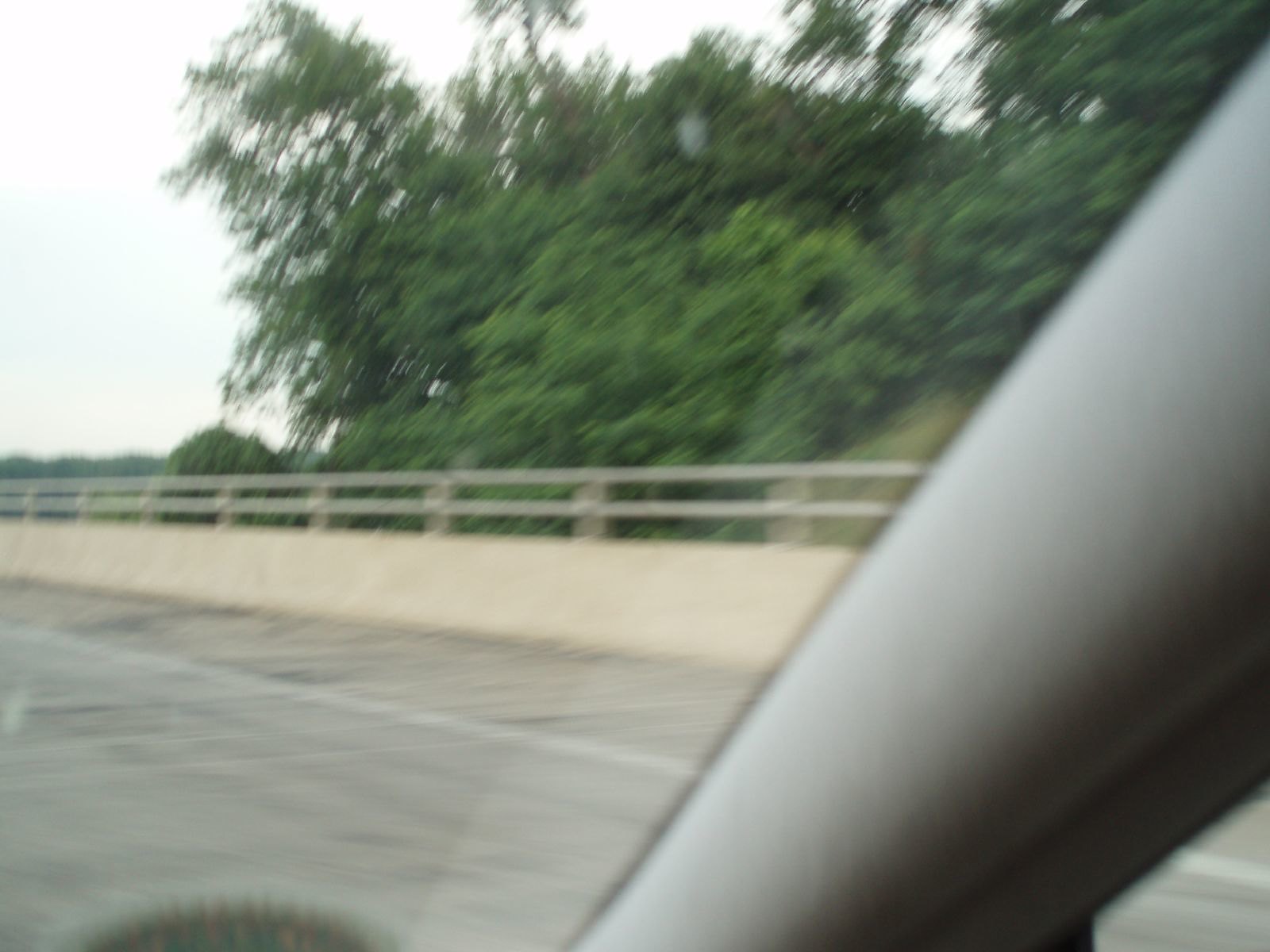This photograph captures a view from inside a moving car, likely taken from the front passenger seat. Through the windshield, the side of a road is visible, characterized by a solid white wall and double guardrails. Large, green trees loom behind the barriers, under a grey, overcast sky. The road appears to be a cement overpass or bridge, distinct from typical asphalt. The image also shows a blurred glimpse of green shrubbery and a concrete barrier with a metal fence that separates traffic lanes. Inside the car, the light grey interior features a long, angled frame with light green upholstery fabric between the windshield and the side window. The metal frame of the window is a cream-colored beige, adding to the interior details. The blurriness of the photo suggests that the car is in motion. The abundance of leaves on the trees indicates that the season might be spring or summer.